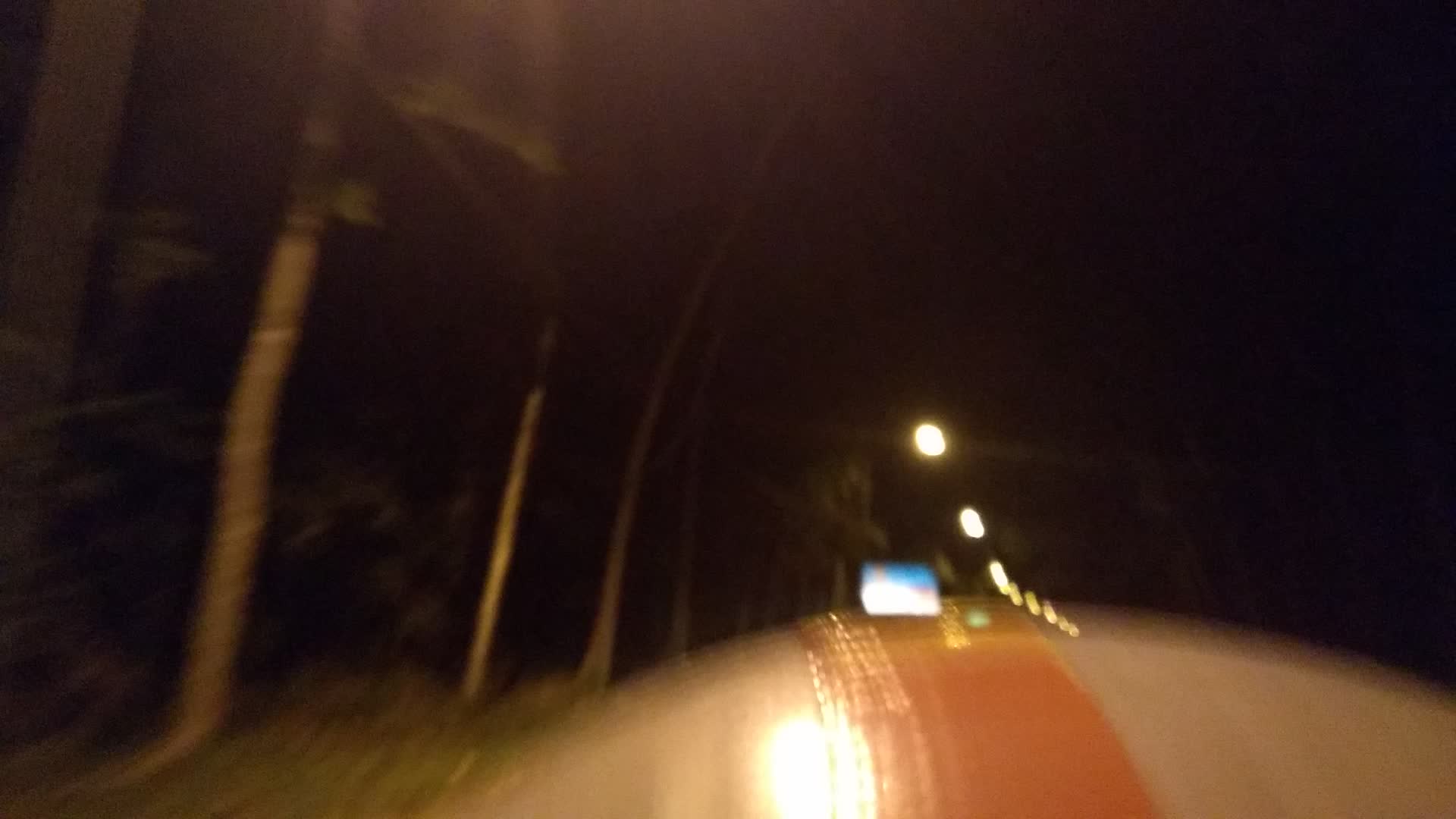The image captures a nighttime outdoor scene with a dark, black sky overhead, indicative of the late hour. The foreground reveals a slick road, which appears gray and brown, adding to the eerie ambiance of the setting. Tall, thin trees and overlapping branches loom on both sides of the road, though the image is somewhat blurry, especially toward the right side where the trees blend with the unpredictable texture of leaves scattered at the bottom. Off in the distance, there's a trail of yellow and white circular lights, possibly streetlights, giving the impression of poles that are just out of clear view. These lights create an array of reflections that might be from a windshield, enhancing the sense of depth and distance. Toward the lower part of the photograph, there is a distinct, circular object with a red stripe and a white border, which could be mistaken for a street sign due to its reflective nature. The entire scene has a haunting, almost cinematic quality, with the overlapping trees lending it a foreboding, almost surreal atmosphere.